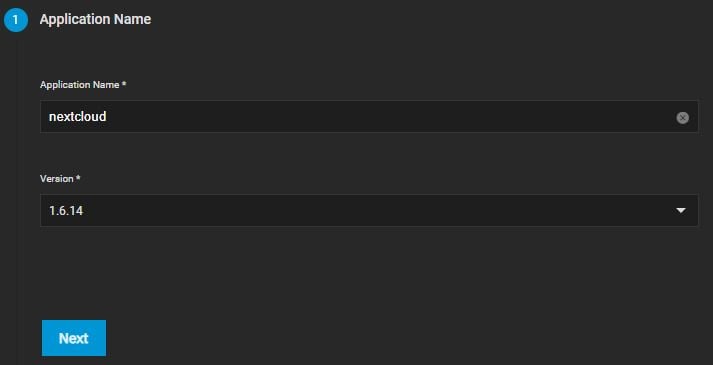The image depicts a web application setup page. At the top of the page, there is a blue circular icon with the number "1" in white, accompanied by the text "Application Name." Below this heading, there's a field labeled "Application Name" marked with an asterisk, indicating it is a required field. Within this field, the text "Next Cloud" appears in white, and there is a gray "X" button to clear the input if needed.

Further down, the page features another field labeled "Version," also indicated as mandatory with an asterisk. This field displays the version number "1.6.14" and includes a drop-down arrow, suggesting that the user can select or change the version number from a list of options.

At the bottom of the page, there is a single interactive element: a sky-blue button with the word "Next" written in white. This button allows users to proceed to the next step in the setup process. The overall background of the page is a blend of gray and black, with white text predominantly used for clarity, while blue icons highlight specific elements, adding a touch of color.

The page serves as an initial setup interface for configuring an application, allowing for the input of an application name and version. The layout and design, featuring navigation elements like a drop-down menu and a next step button, suggest that it is part of a web-based application setup or settings module.